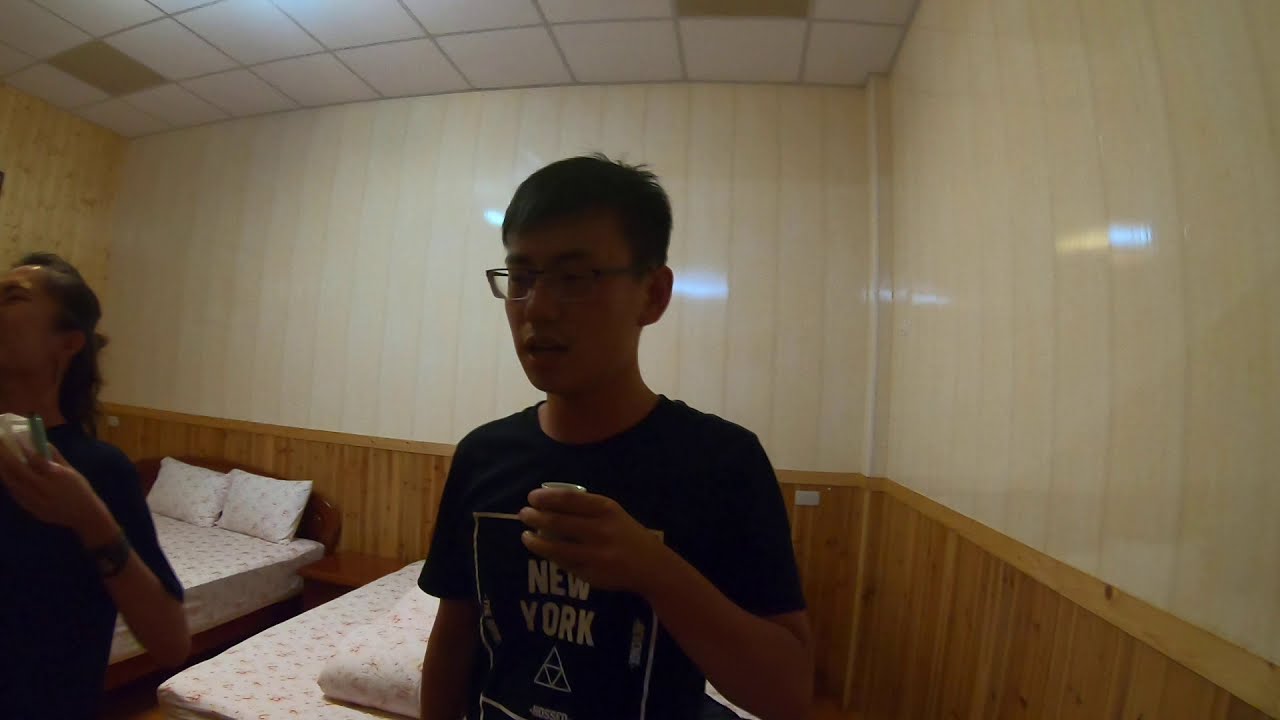In this dimly lit indoor photograph, we see a young man of Asian descent with black hair and glasses, standing in a small room. He is wearing a black crew-neck t-shirt that prominently displays the words "New York" in white capital letters, framed by a white rectangular border underneath which there is a white triangle. His left arm is bent at the elbow, holding a small white cup, possibly a sake cup, at chest height. He appears to be speaking, as his mouth is slightly open. The room around him features glossy beige walls with wooden panels along the bottom half and white ceiling tiles above. Behind him, two beds with white sheets adorned with pink floral patterns and matching pillows are visible. An older Asian woman with black hair, also wearing a black t-shirt, stands partially visible to his left, holding an indistinct object. The photograph's poor lighting casts shadows and highlights the reflective surfaces of the walls and ceiling, but fails to illuminate the subjects clearly.